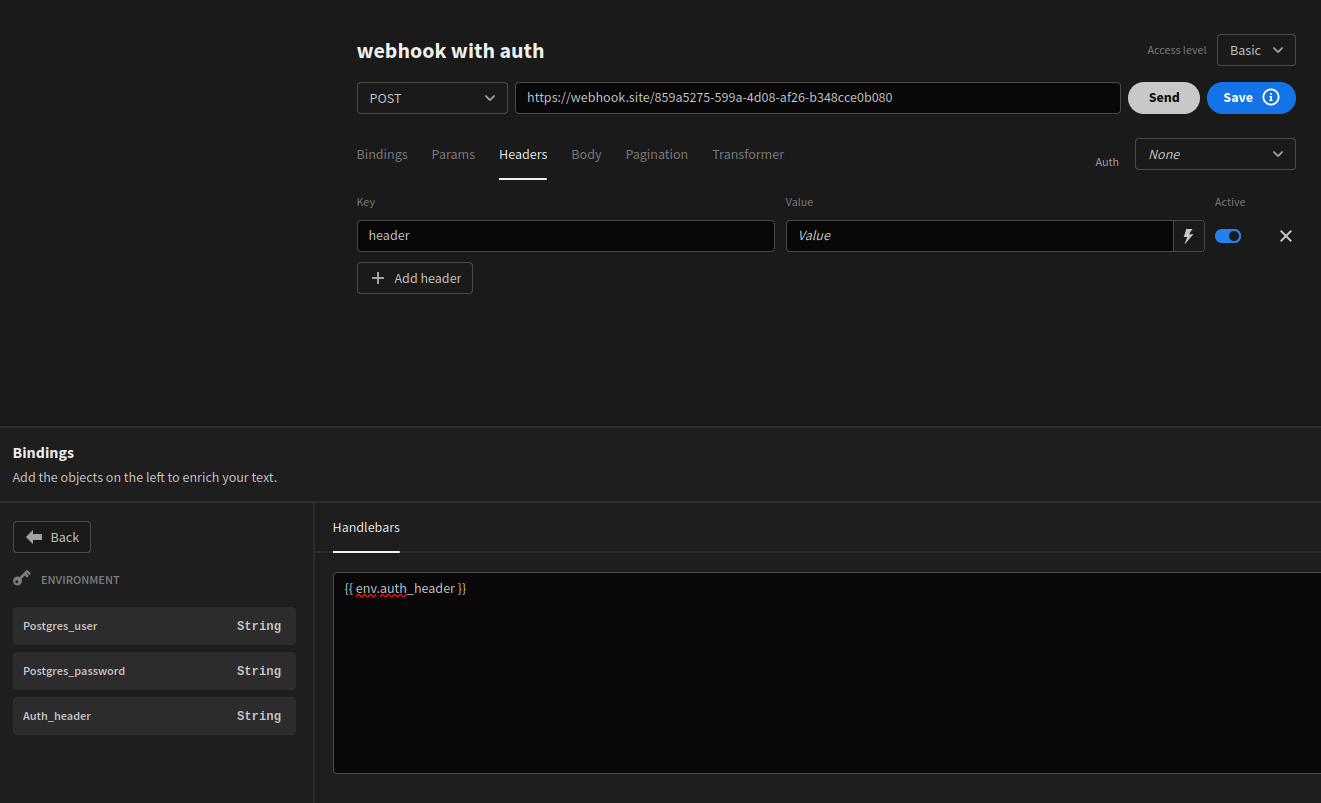The image displays a detailed printout of a webhook interface with an authorization form. Here's a breakdown of its elements:

Starting at the top, there is a section labeled "Webhook with Authorization," indicating that the access level is "Basic." Just below this, you can identify a "POST" method followed by a URL, `webhook.site/[the address]`. Accompanying the URL are two buttons: a white "Send" button on the left and a blue "Save" button to the right.

Moving to the next section, a series of tabs are listed: Bindings, Params, Headers, Body, Pagination, Transformer, and Authorization. The "Headers" tab is currently active, as indicated by a white underline.

Within the Headers section, there is a table-like format with two columns labeled "Key" and "Value." The first row reads "Header" under the Key column and "Value" under the Value column, with an active blue indicator button situated next to an X, suggesting the ability to delete this entry. Below this row, there is an option to add more headers.

At the bottom of the printout, there is additional information in white text. From left to right, it reads: "Bindings: Add the objects on the left to enrich your text, with a back button to navigate." There is also mention of an environment key, including details like "Postgres User String," "Postgres Password String," and "Authorization Header String."

Prominently featured near the bottom center is a section dedicated to "Handlebars," displaying an ENV authorization header. This is highlighted with red squiggly lines, indicating an error or issue that needs attention. 

Overall, the image meticulously outlines the structure of a webhook authorization form, highlighting various sections and functionalities crucial for setting headers and managing authorization.